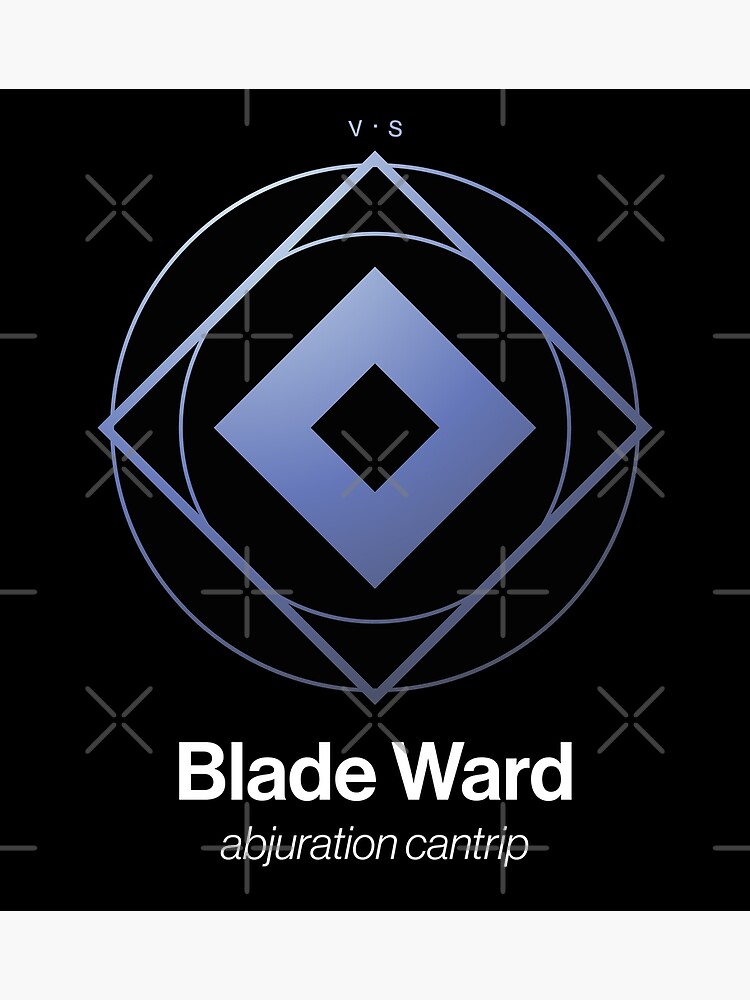The image features a logo-like design with a complex layout and muted colors. At the center, there is a small diamond-shaped figure with four corners, rendered in a light blue-silverish hue. This central diamond is surrounded by a thin lined circle of the same light blue-silverish color. Encircling this is a much larger, thin-lined diamond, at the edges of which are additional thin-lined circles located just inside the tips of the larger diamond. The entire geometric arrangement shares a consistent bluish-silver palette.

Above this intricate design, the text "V.S." is displayed in very thin white letters. Immediately below the geometric shapes, the white text reads "Blade Ward," followed by "Abjuration Cantrip." The background is primarily black and is overlaid with a subtle watermark consisting of faint gray crosses and X’s. The overall effect suggests a carefully constructed logo, possibly representing a company or a specific product.